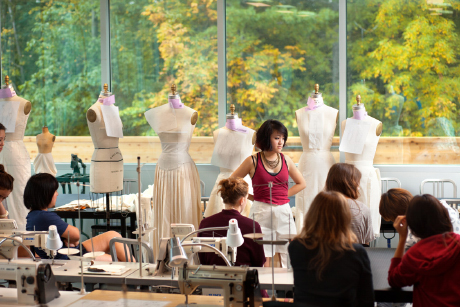In a room filled with natural light streaming through large glass windows, which offer a serene view of a lush green forest with yellow and light green leaves, a group of women are seated at sewing machines, attentively listening to an instructor. The instructor, possibly of Asian descent, stands at the front wearing a red tank top paired with a white skirt, and a necklace. Behind her, a line of headless mannequins in various stages of dress stands in front of the windows. The mannequins display different designs, contributing to what appears to be a fashion design classroom. Additional sewing machines and seated individuals, likely students, are visible in the background, further emphasizing the educational setting where participants are presumably working on or conceptualizing dress designs.